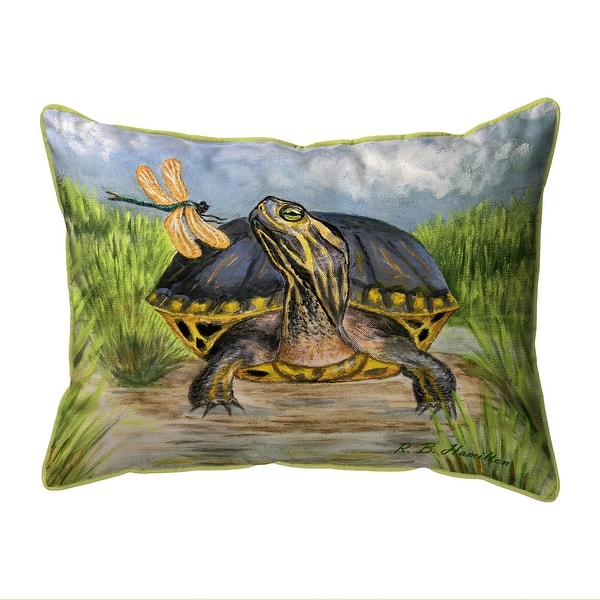This image depicts a rectangular pillow with a vibrant canvas print, framed by lime green piping around the edges. The background of the print features a serene blue sky with occasional white and gray clouds at the top. The scene is set in a marshy swamp, enriched with patches of green, leafy plants and brown, wet ground that suggests a typical habitat for turtles. In the center of the pillow dominates a painted turtle, whose head is slightly raised and pointed towards the upper left. The turtle boasts a black shell adorned with yellow dots around the rim, while its underside is a darker gold with black markings. The turtle's face is characterized by striking black and yellow stripes and a green eye, and its spiky claws are clearly visible. By its head, a dragonfly with teal-blue and perhaps light orange wings, and a green body, appears to hover, adding a dynamic element to the composition. The earthy and aquatic tones of the background are complemented by the artistic rendering of the turtle and the insect. There is also a delicate green outline near the pillow's bottom, giving it a distinct finish. The lower right corner is signed with "RV Hamilton."